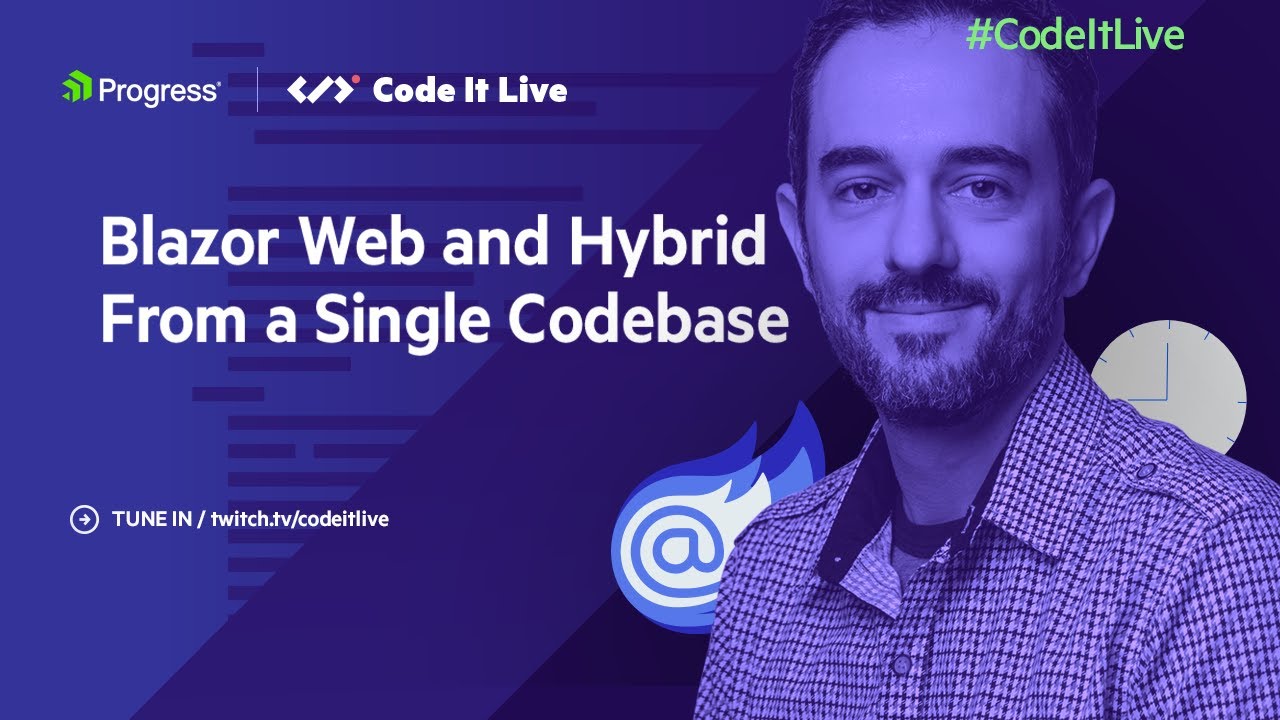This image is likely an advertisement for "Code It Live". The background is a royal blue color, giving the overall image a vibrant and modern feel. In the upper right corner, "#CodeItLive" is prominently displayed in green text. The upper left corner features the word "Progress" in white print. Next to this, there is an icon incorporating a stylized "C" and a backwards "L" representing "Code It Live."

Beneath this icon, a tagline in white text reads, "Blazor web and hybrid from a single code base." A smiling man is centered in the image, although the blue background casts a blue hue onto his skin. Despite this, his dark hair, eyebrows, probable brown eyes, and facial hair are clearly visible. He is dressed in a plaid shirt, adding a casual touch to his appearance.

At the bottom of the image, viewers are invited to "Tune in at twitch.tv/codeitlive," encouraging engagement with the "Code It Live" programming community.